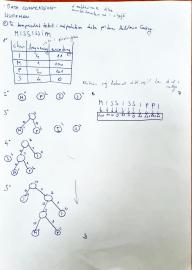This indoor close-up color photograph captures a small piece of vertically oriented white paper. The paper is printed in blue ink and appears to be notes, likely for a biology or chemistry class. In the upper-left corner, handwritten text is visible, running from left to right. Below this, a grid comprising three columns and five rows contains various letters and markings. The small size of the image renders the text illegible, even when magnified. On the bottom left side of the page, a collection of circles connected by vertical lines is visible, resembling diagrams of molecular structures, with numbers inside the circles indicating simple chemical bonds or elements. Along the left column, rows are numbered, suggesting this could be a quiz or an exercise sheet where answers were recorded. However, due to the fine print, the specific content remains unreadable.